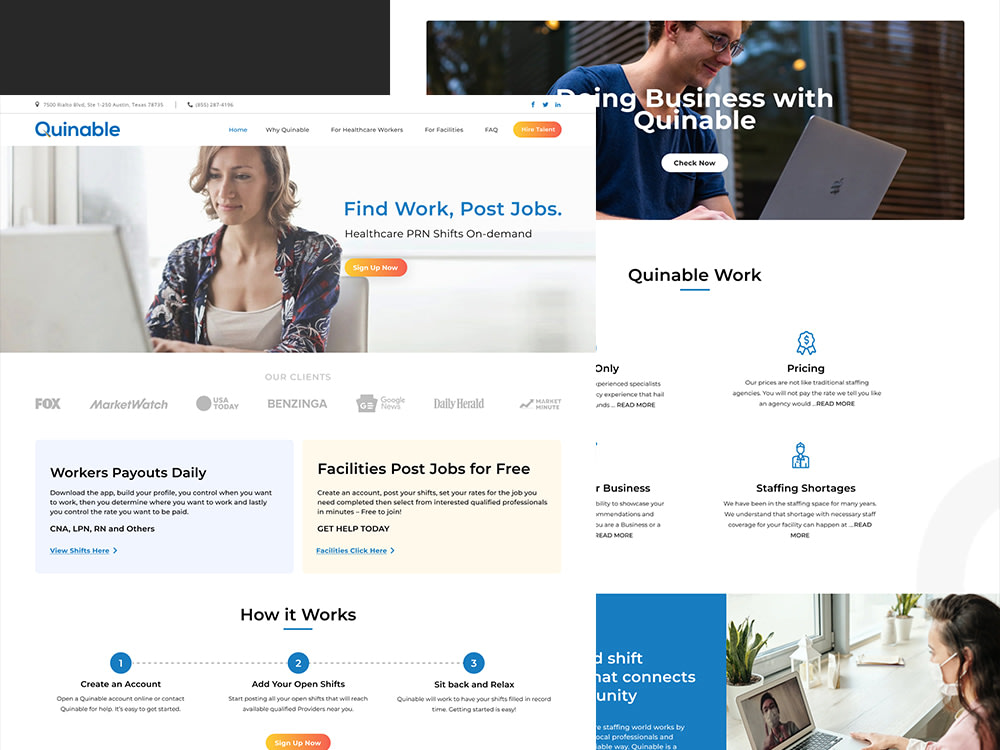The screenshot showcases the homepage of a website called "Quinable" (Q-U-I-N-A-B-L-E). The layout features a clean, white background with a blue and gold theme. On the left side of the page, the site’s logo "Quinable" is prominently displayed in blue text. A horizontal navigation menu follows, listing options from left to right: "Home," "Why Quinable," two unreadable items, "FAQ," and a gold call-to-action button with rounded edges saying "Sign Up Now" in white text.

Beneath the menu, there is an image of a white woman with blonde hair just above shoulder length, working on a silver-gray laptop. She is wearing a dark blouse with abstract designs and a light gray, low-cut shirt underneath. To the right of this image, in blue font, the words "Find Work Post Jobs" are visible. 

On the upper right corner of the page, partially hidden, is the text "Business with Quinable." Accompanying this text is a photo of a white man with dark-framed glasses wearing a dark blue T-shirt, also working on a gray laptop.

Centrally located on the page are two key phrases: "Workers Pay Out Daily" and "Facilities Post Jobs for Free," indicating the website’s purpose as a job search and job posting platform.

In the lower left corner, the text "How It Works" introduces a three-step process, each step numbered within a blue circle. Step 1: "Create an Account," Step 2: "Add Your Open Shifts," and Step 3: "Sit Back and Enjoy."

Finally, in the lower right corner, there is another image of a woman wearing a surgical mask while sitting at a computer with a screen displaying another woman also in a surgical mask. This image further emphasizes the practical, real-world applications of the website.

Overall, this well-organized layout clearly introduces Quinable as a job search and job posting platform designed for both businesses and individuals.